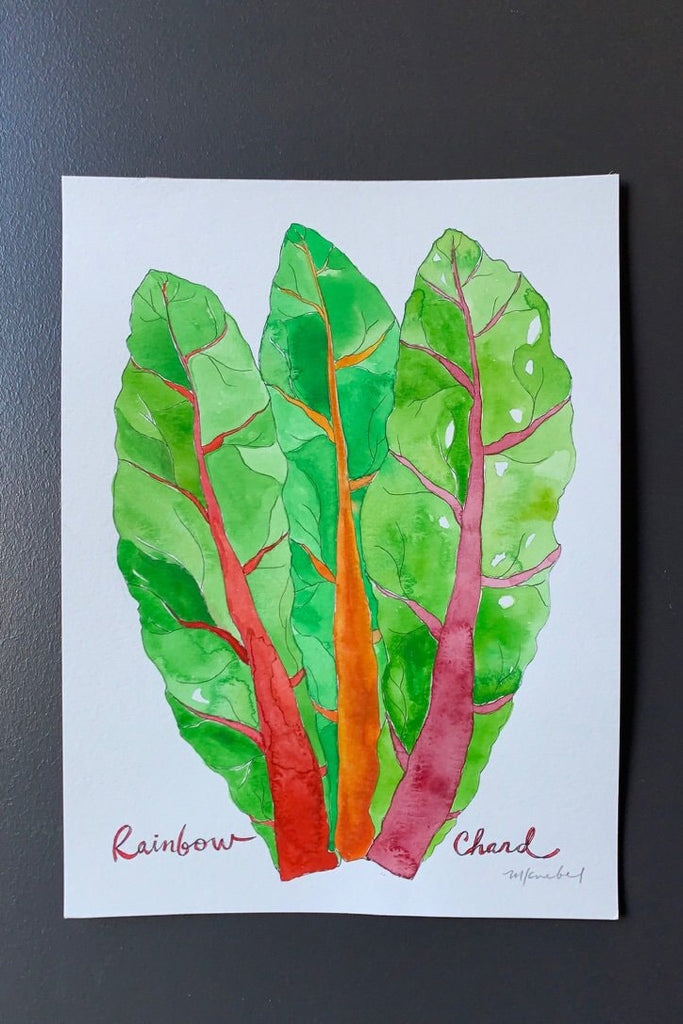This detailed watercolor illustration depicts three vibrant leaves of rainbow Swiss chard arranged in a playful composition against a stark black background. Each leaf, tall and elliptical with pointed tips, features a vivid green hue with colorful veins branching out in intricate patterns. The leaf on the left, angled slightly toward the top left corner, showcases a prominent red central vein. The central leaf, partially obscured by the first, exhibits a bold orange vein and points upward towards the center of the frame. The leaf on the right overlaps the central leaf, angling towards the upper right, with a distinctive purple central vein. The word "rainbow" in elegant red cursive graces the left edge of the illustration, while "chard" in matching maroon cursive is scripted on the right. This artistic piece, signed with an illegible black signature in the bottom right corner, is painted on a piece of white paper and mounted against a black wall, emphasizing the vibrant colors and delicate details of the rainbow chard leaves.